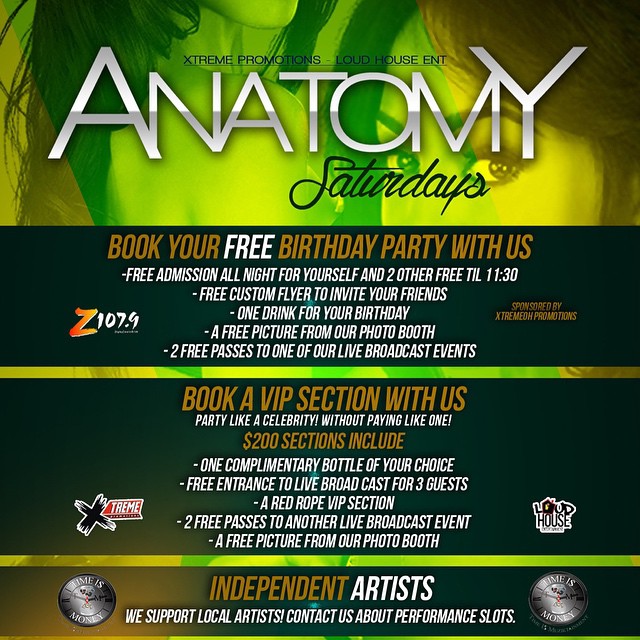This eye-catching advertisement features a vibrant mix of green hues and promotes "Anatomy Saturdays" by Extreme Promotions and Loud House ENT. The top section, set against a subtly visible background of two women's shoulders, eyes, and hair, announces the event with bold typography: "Extreme Promotions, Loud House, ENT" in black, followed by "ANATOMY" in large silver capital letters and "SATURDAYS" in black cursive.

The subsequent section, framed by a dark green background, invites you to "BOOK YOUR FREE BIRTHDAY PARTY WITH US" in tan and white text. This offer includes perks like "FREE ADMISSION" and "ONE DRINK FOR YOUR BIRTHDAY."

A lime and yellow dividing line leads to another rectangle, where "BOOK A VIP SECTION WITH US" promises star treatment for $200, including a complimentary bottle of your choice and free entry for three guests to another live broadcast event.

At the bottom, a green rectangle highlights "INDEPENDENT" in tan and "ARTIST" in white, encouraging local artists to contact for performance slots.